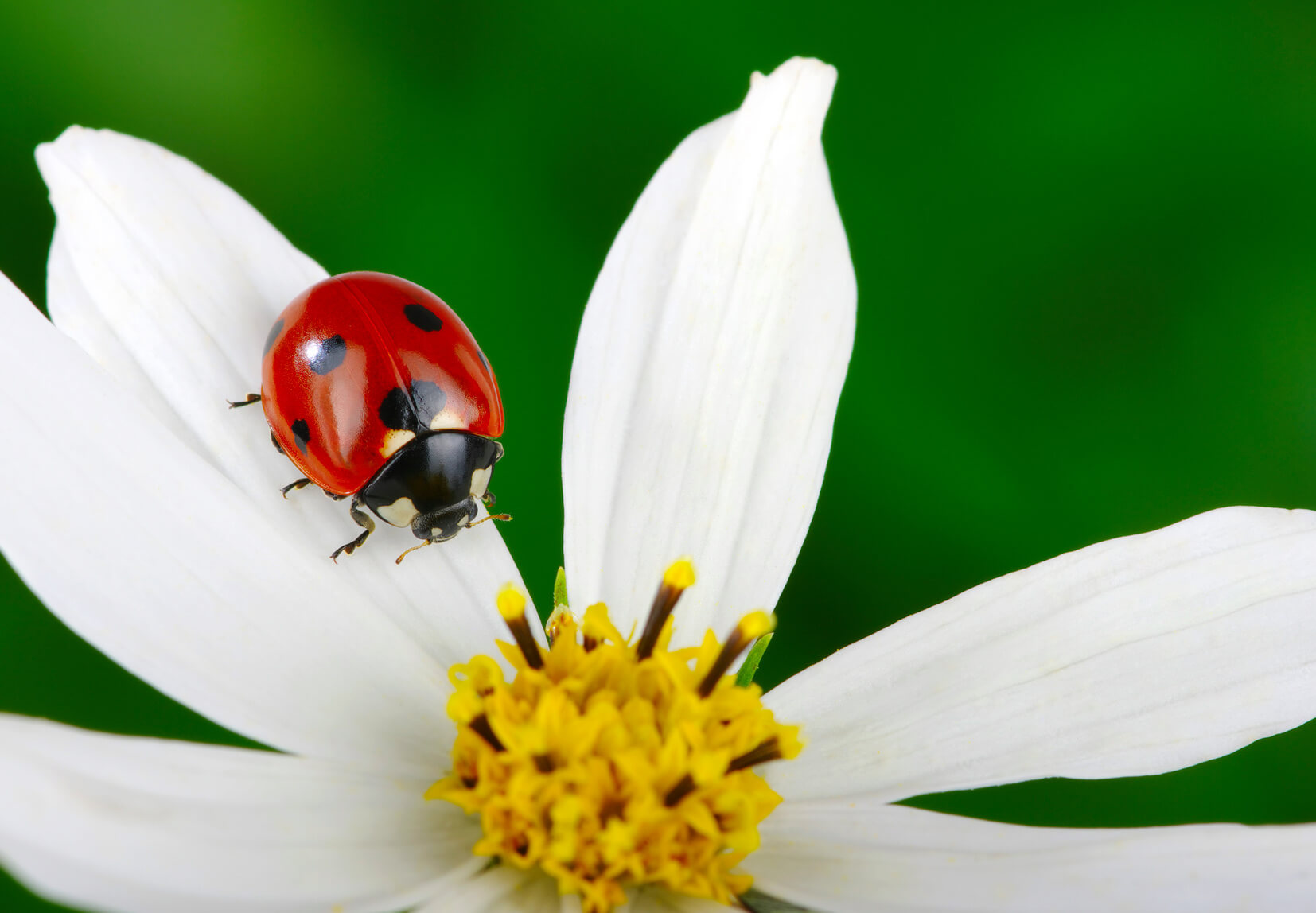This captivating full-color photograph, an artistic nature shot likely taken on a sunny day, showcases a vibrant scene featuring a striking red ladybug in sharp focus. The ladybug, with six black spots on its shiny back, two white spots on its midsection, and two more on its head, is captured mid-climb on a narrow, white petal of a flower. It appears to be making its way towards the bright yellow center of the flower, which is encircled by about six to seven elongated petals. The ladybug's six legs are partially visible, with three clearly seen on one side and one peeking out on the other, alongside its two distinct antennae. The backdrop of the photograph is a lush, green blur, suggestive of vegetation found in a forest or field, providing a contrastingly soft and diffused background that highlights the detailed beauty of the ladybug and the flower. The horizontal orientation of the image without any border frames this serene moment in nature perfectly.